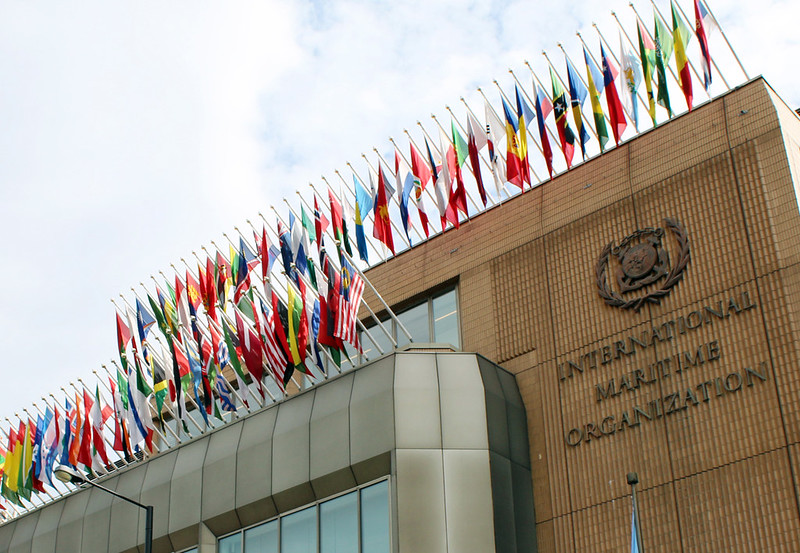This image features the headquarters of the International Maritime Organization, as indicated by the bold letters and organization’s logo displayed prominently on the building’s front. The building showcases an interesting architectural contrast: while the main structure is classical and brown, likely made of wood or brick with numerous windows, a modern, silvery metal protrusion extends from its front, featuring large windows. Several flags adorn both the main building and the protruding part, including those of Jamaica, the United States, and the United Kingdom, although most are unidentifiable. A street lamp stands in front of the structure. The background appears stark white, suggesting either a cloudy sky or an overexposed photograph, and the bottom portion of the building and any entrances are not visible in the frame.